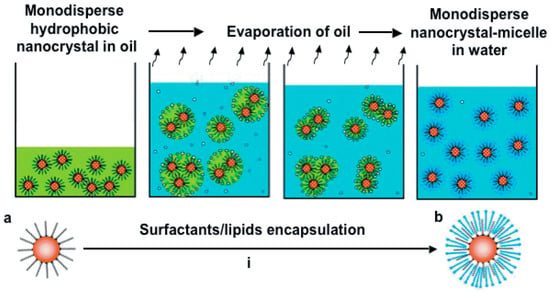The image is a detailed scientific diagram illustrating the transformation of monodisperse hydrophobic nanocrystals in oil to monodisperse nanocrystal micelles in water. At the bottom of the diagram, there is a cell or organism labeled 'A', depicted with orange circles and black lines, representing the initial stage. This cell undergoes a process called surfactants/lipids encapsulation, highlighted by a horizontal black arrow pointing to 'B', where the cell is larger with blue lines signifying the final stage.

The top section comprises four sequential images. The first image shows a container with a green liquid labeled "monodisperse hydrophobic nanocrystal in oil," containing orange circles with black lines. The second and third images, marked by arrows indicating "evaporation of oil," depict the transition where the orange circles become slightly modified, surrounded now by an aqua-blue liquid. Finally, the fourth image, under the label "monodisperse nanocrystal micelle in water," shows the fully transformed state of the nanocrystals as orange circles with blue lines in aqua.

Overall, the diagram meticulously traces the metamorphosis from initial monodisperse hydrophobic nanocrystals encapsulated in oil to their final state as micelles in water, emphasizing the encapsulation process and highlighting the stages with specific visual cues and descriptive labels.